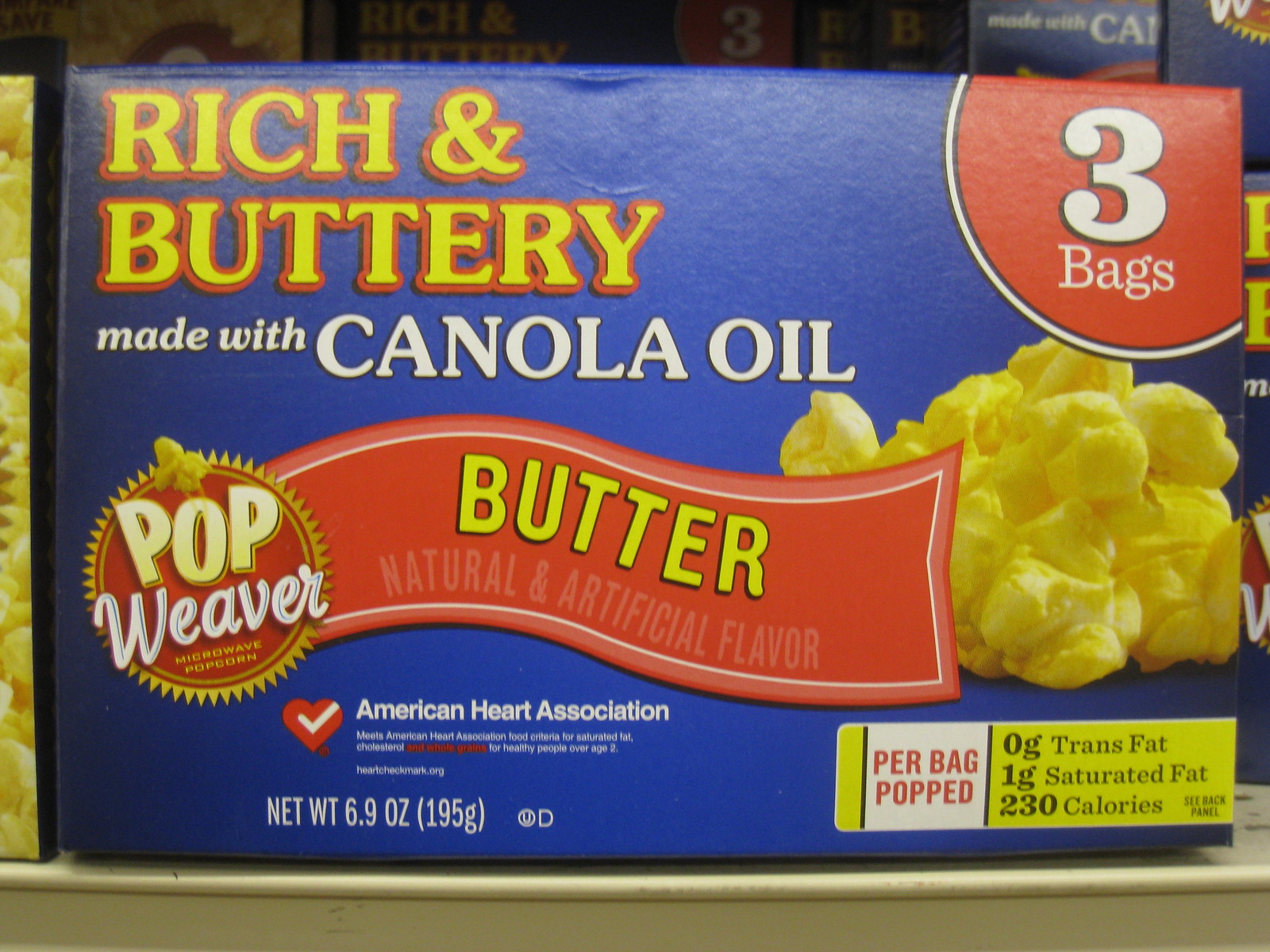This image features a prominently displayed package of Pop Weaver popcorn on a store shelf, surrounded by identical boxes in the background. The box itself is a vibrant blue rectangular prism, adorned with rich visual details. At the top left corner, bold yellow and red type spells out "Rich and Buttery." In the top right, a vivid red semi-circle declares "Three Bags" in white text, accentuated by a black border. Centered on the box, the phrase "Made with Canola Oil" stands out in all caps, slightly bolded and written in white.

The lower section of the box showcases a ribbon-like graphic in red, stating "Butter" in yellow with a note on natural and artificial flavor. An image portraying approximately 10 to 12 popped popcorn kernels, vividly yellow, adds a touch of realism to the package design. Nutritional information is meticulously provided in a section highlighted by a white background with red and black text, specifying "Per Bag Popped: Zero Trans Fats, One Gram Saturated Fat, 230 Calories."

The left side of the box features a red heart with a white check mark, accompanied by the American Heart Association logo and text, also written in white. Finally, the lower right corner confirms the net weight of the package: 6.9 ounces (195 grams), again detailed in white text for clarity. The overall design artfully combines functionality with an eye-catching presentation, making it an appealing choice on the grocery shelf.